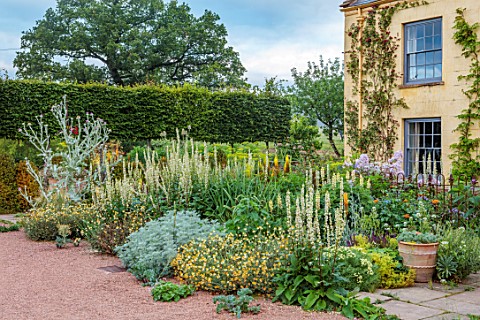In this image, we see the front yard of a two-story, yellow building with a lot of greenery and colorful flowers. The building, situated on the right side, features two large windows and has a rain gutter running from the roof to the ground. Ivy and other plants climb up the façade of the building, adding a lush touch to the otherwise plain wall. The foreground is filled with a variety of plants and flowers, including yellow, white, and purple blooms, as well as leafy plants and tall beige cattail-like structures. There is also a pot with plants on the right side. The ground near the front corner on the left is covered with red rocks or gravel. Densely packed bushes and a prominent large tree are visible in the background, set against a clear blue sky.